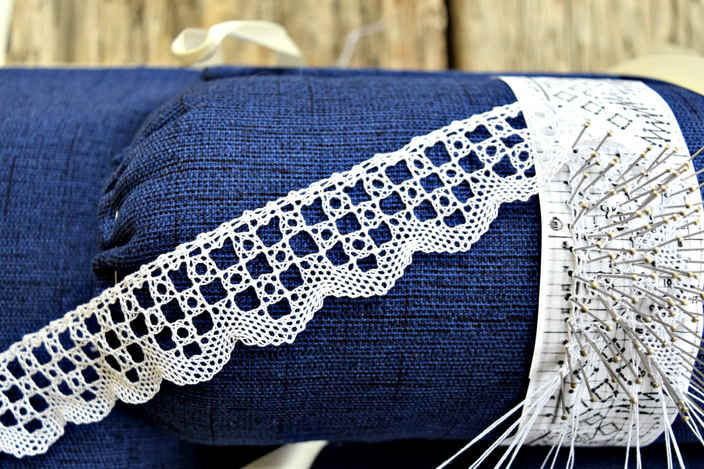The color photograph provides an overhead view of an intricate lace-making process, set on a dark blue bolster pillow, which at first glance may resemble a couch cushion or sofa. To the left, a band of meticulously crafted lace, composed of fine white thread, showcases the intricate skill involved. The right side of the image reveals the ongoing work, with nearly a hundred pins securing the developing lace pattern. Each pin has threads intricately wound around it, guiding the creation of the lace. The scene features thin, nail-like pins that assist in the threading process, providing a detailed glimpse into this traditional craft. The overall composition and background suggest the setup is possibly on a piece of blue upholstery, such as a sofa or a couch, adding a familiar, homey context to the meticulous artisan’s workspace.